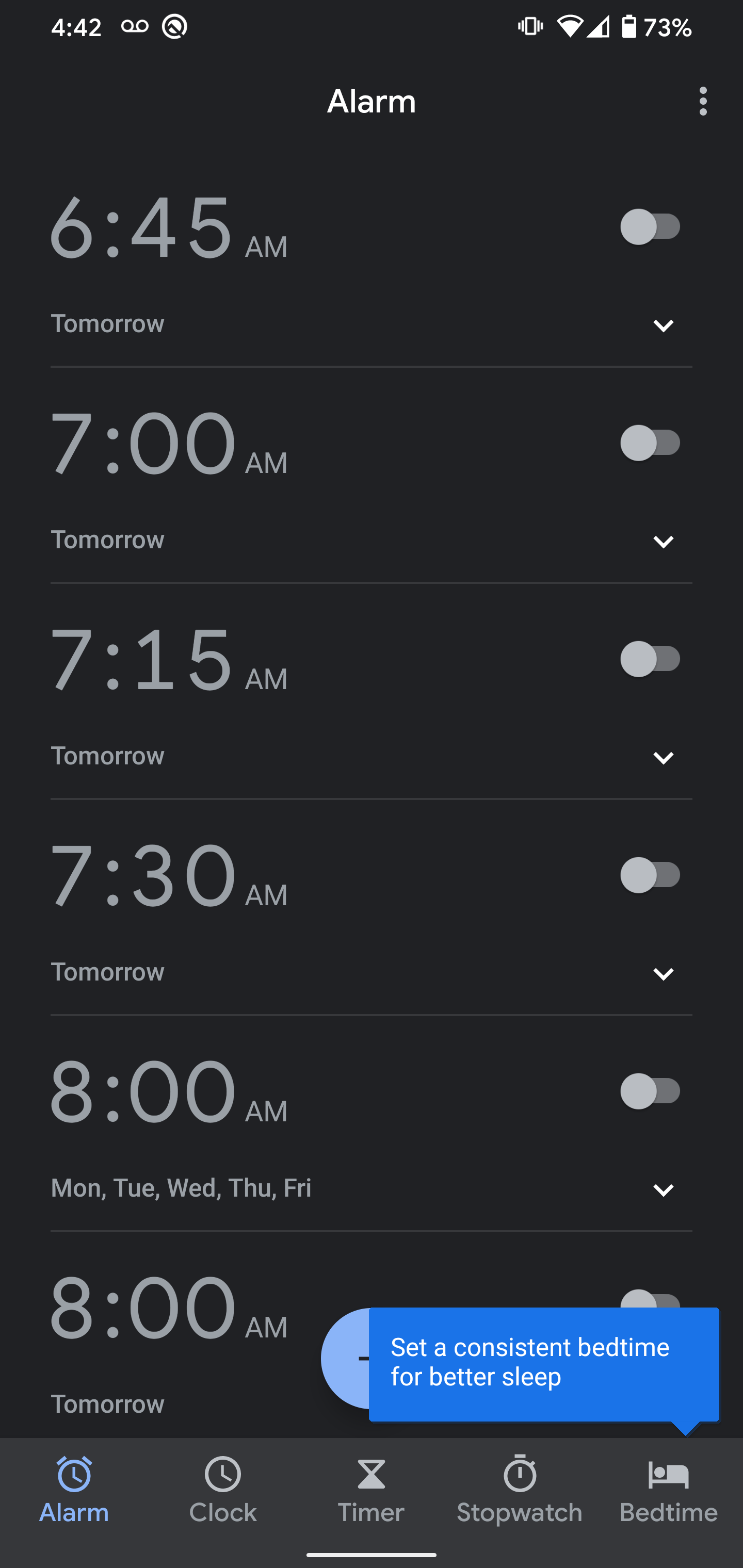The image displayed on a cell phone screen shows a detailed overview of the alarm settings. The battery life indicator reads 73%, and the phone has a strong network connection. The current time displayed is 4:42 PM. This screen, specifically the alarm section, lists several alarms that are all set to off:

1. 6:45 AM with a note "Tomorrow" - Off
2. 7:00 AM "Tomorrow" - Off
3. 7:15 AM "Tomorrow" - Off
4. 7:30 AM "Tomorrow" - Off
5. 8:00 AM on weekdays (Monday to Friday) - Off

There is also a highlighted message in a blue box stating, "Set a consistent bedtime for better sleep." 

At the bottom of the screen, there are navigation options identified by text and icons for different functionalities: Alarm, Clock, Timer, Stopwatch, and Bedtime. The alarm option is highlighted in blue, signifying it is currently active. Each option has an icon above it in white except for the Alarm, which also has a small white line beneath it, indicating selection. Each alarm entry has a light gray line underneath it, and drop-down arrows are present for additional settings or options for each alarm.